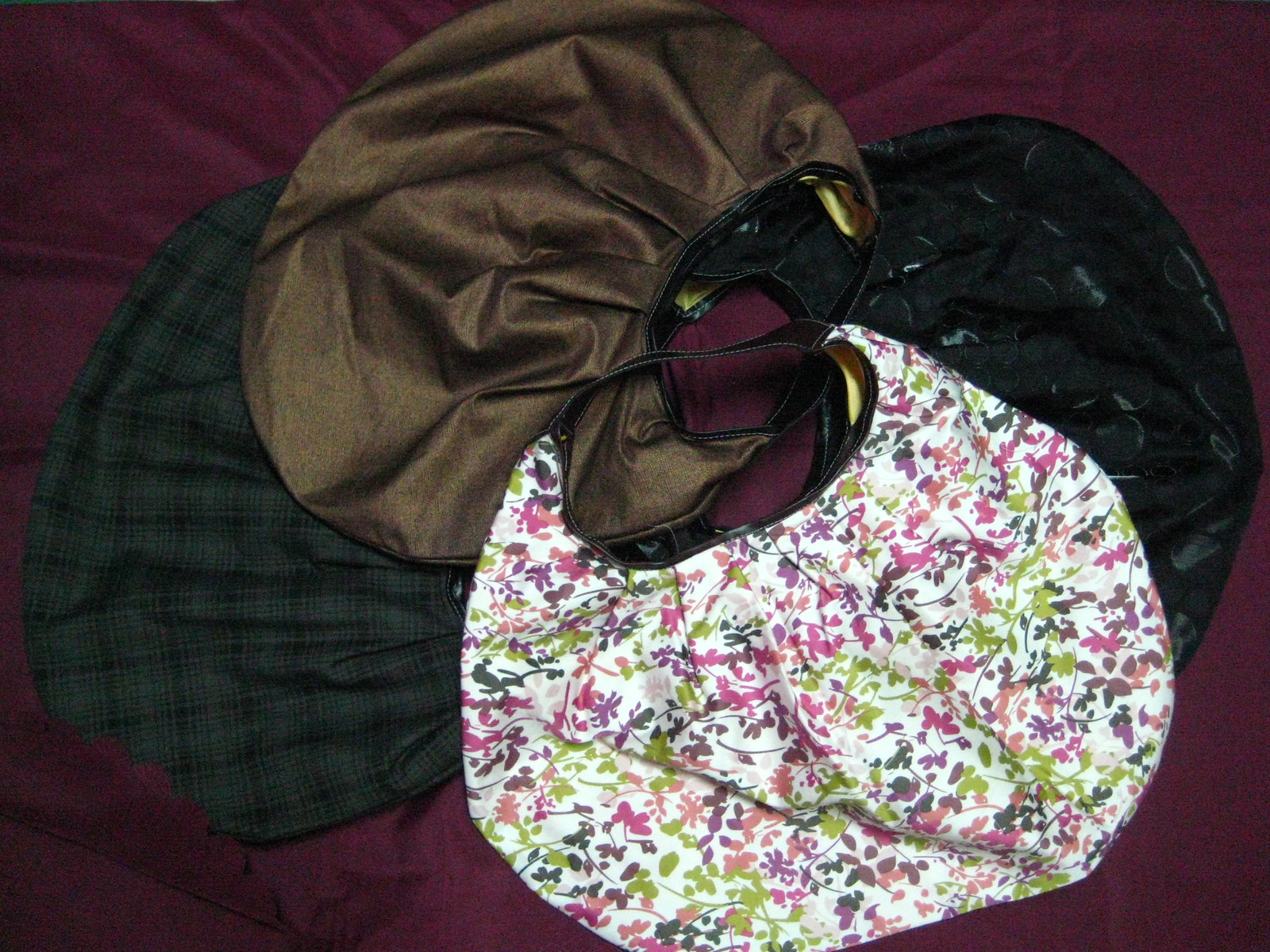This image captures four distinctly styled yet identically shaped handbags arranged in a circular pattern on a maroon fabric background, which displays slight wrinkles. The focal handbag, situated on top, features a white base adorned with a vibrant floral pattern in shades of purple, pink, and green, complemented by a black handle with white stitching. To its right and underneath it lies a black purse with a subtle brocade design, possibly indicative of a luxury brand. The third purse, made of bronze-colored material, also includes a black handle, while the fourth handbag, partially visible underneath, displays a dark green and black plaid pattern. The arrangement of the bags, overlapping with their handles intertwining, showcases a harmonious blend of textures and hues against the richly colored backdrop.